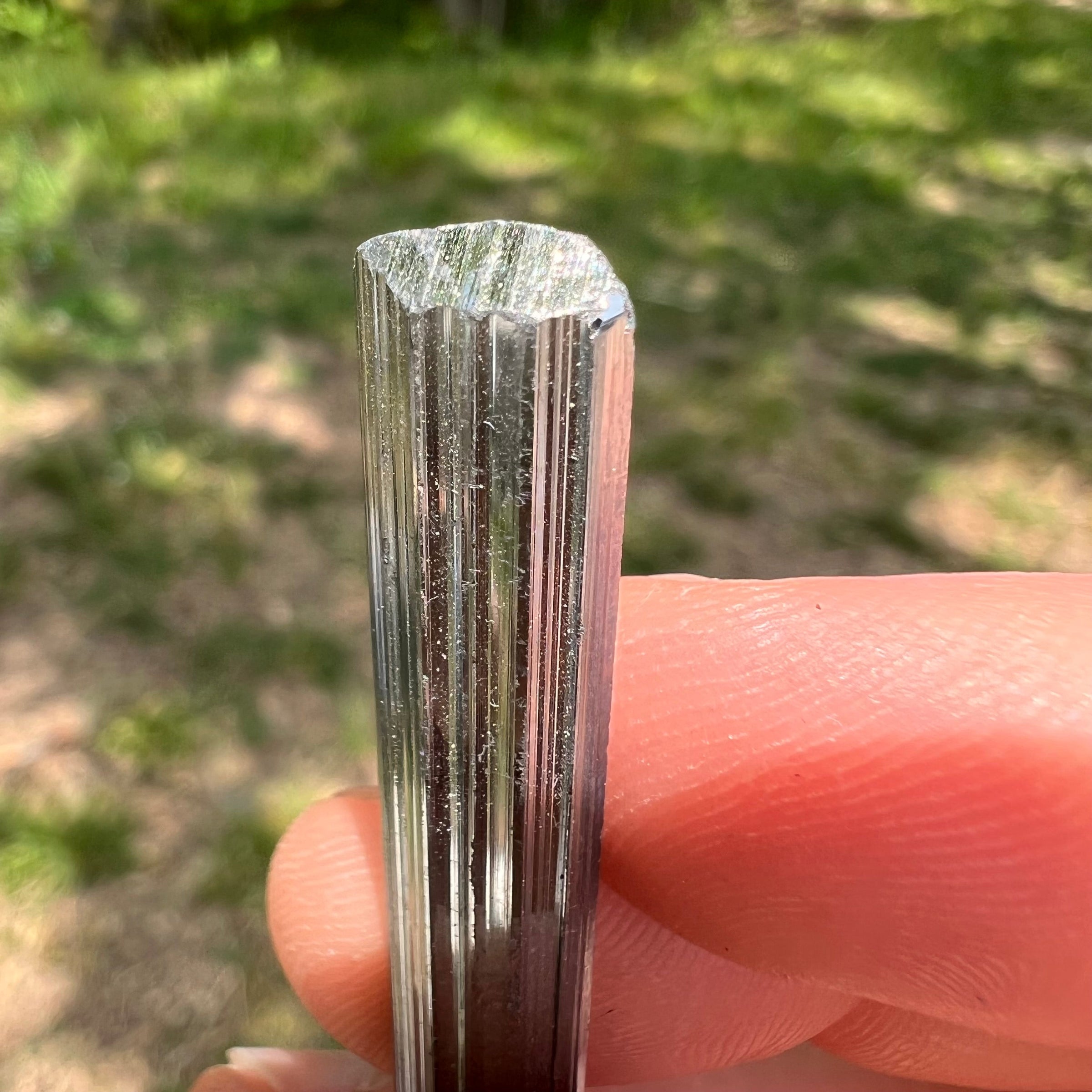This is a high-resolution, close-up image of a shiny, metallic object, likely a silver-colored bar. Every striation, imperfection, and small scratch on the object's surface is clearly visible, with significant detail captured, especially towards the top where it appears to be chipped, revealing additional grooves and breakage marks. The reflective nature of the metal allows for the fair-skinned, rosy-tinted fingers of the person holding it to be seen mirrored on its surface. The object comes into the image from the bottom middle and extends upwards past the center, its bends and curves giving off black and silver hues with slight bluish tints towards the end. The person's fingers, positioned in the lower right quadrant and at the middle bottom of the image, show all their ridges due to the proximity. The background features vivid green grass with some out-of-focus brown areas, providing a natural setting for the metallic object.